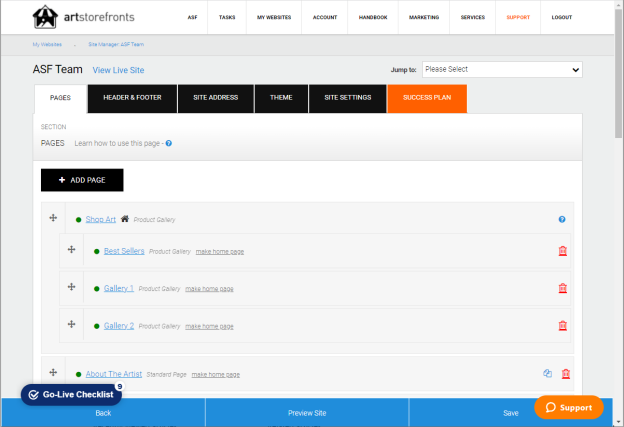This image is a detailed screenshot of the interface for the ArtStorefronts application, presented as a single word. At the top of the interface, the ASF Team section is highlighted, with options to either "View Live Site" or access a dropdown menu containing additional navigational choices, albeit these specific options are not clearly visible in the screenshot.

Currently, the "Pages" tab is selected, showcasing a structured list of different page options such as "Gallery 1," "Gallery 2," and "Best Sellers." Adjacent to this tab are several others: "Header and Footer," "Address," "Theme," "Site Settings," and a "Success Plan." Below the list of existing pages, there is an "Add a Page" section, allowing users to expand the site's content further. Each page entry is accompanied by a small plus sign, indicating the availability of expandable details.

For users who might find the interface overwhelming, a prominent yellow or orange support button with a chat bubble icon is located at the bottom right corner of the screen. On the lower left side, there is a "Go-Live Checklist" option to assist users in launching their site. The very bottom of the screenshot reveals additional options, but these are unreadable due to poor image resolution.

This comprehensive depiction of the ArtStorefronts interface demonstrates an array of available tools and navigational elements designed to assist users in managing and customizing their webpages.